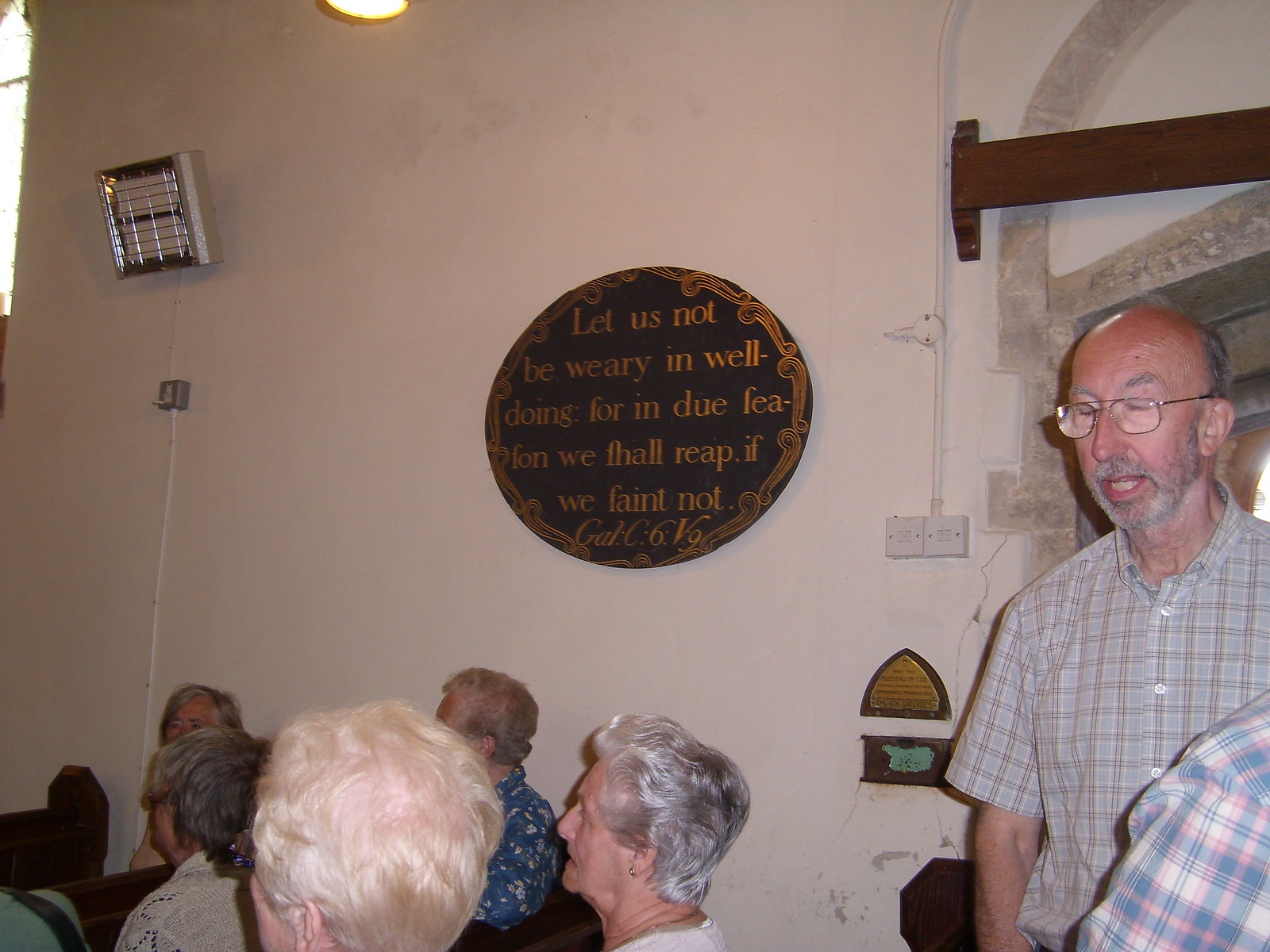The image depicts an interior scene of a church or fellowship hall, characterized by white walls adorned with a circular plaque inscribed with a Bible verse from Galatians 6:9: "Let us not be weary in well-doing, for in due season, we shall reap if we faint not." The setting includes elderly people seated in wooden pews or booths. At the bottom left, the heads of about four elderly women are visible, while on the right side, an elderly man with his mouth open, possibly singing or talking, wears a checked shirt in subtle, beige or light blue tones. Another man, adorned with glasses, a balding head, a beard, and a plaid collared shirt, is captured walking through a doorway. The room's colors are muted, with beige, cream, and light blue hues, under soft lighting. A light fixture mounted on the wall adds to the ambiance, enhancing the subdued and contemplative atmosphere of the gathering.